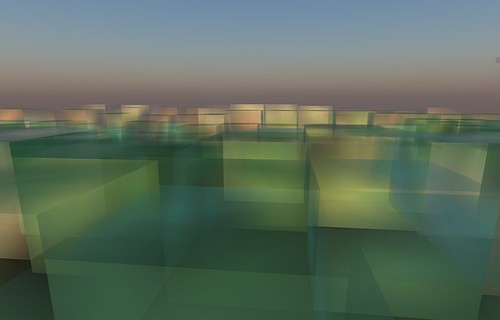The image depicts a digital artwork or painting with a horizontal rectangular shape. It features a vibrant and somewhat blurred cityscape composed of translucent cubes and rectangles of various sizes, arranged to resemble buildings. The cubes are in colors ranging from light brown and green to pink and yellow, creating a virtual space that seems both abstract and structured, with a sense of depth from uneven placements. The foreground of the image starts with blue and bluish-green tones, transitioning to more green, blue, and eventually pink and yellow cubes as they head towards the horizon. The sky above the horizon features a gradient of colors, beginning with a blue at the top, fading to light yellow and pink, and finally darkening to a purplish pink at the skyline. The overall composition suggests a flat and undetailed yet imaginative cityscape, viewed from above, with the cubes representing buildings in a minimalist and translucent style.